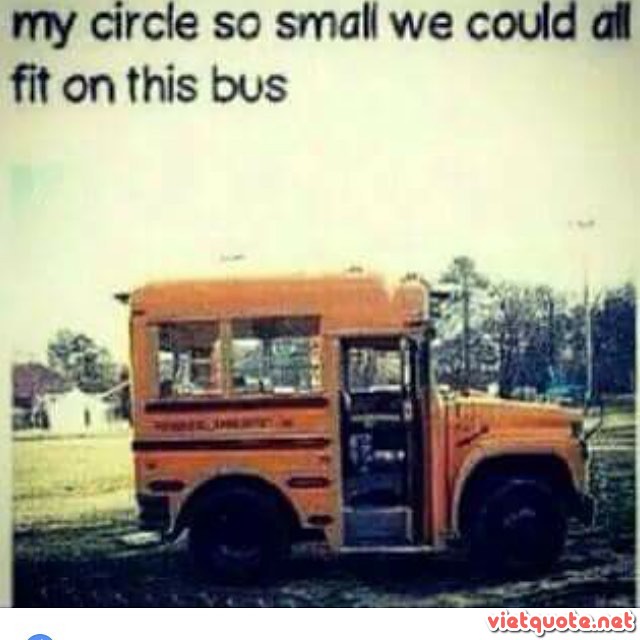This caption encapsulates all the details shared and emphasized across the different descriptions:

A grainy, vintage photograph, possibly taken in the late 70s or early 80s, depicts a tiny yellow school bus, significantly shorter than a standard bus, with just two rows of seats behind the driver's seat. The bus, with its door open, is parked in a grassy field under a blue sky, surrounded by scattered trees, a light pole, and a small white house in the background. Black text at the top of the image humorously declares, "My circle so small, we could all fit on this bus." The photo's low resolution and faded colors add to its nostalgic, worn appearance. At the bottom right, red text reads "VietQuote.net," branding the meme.